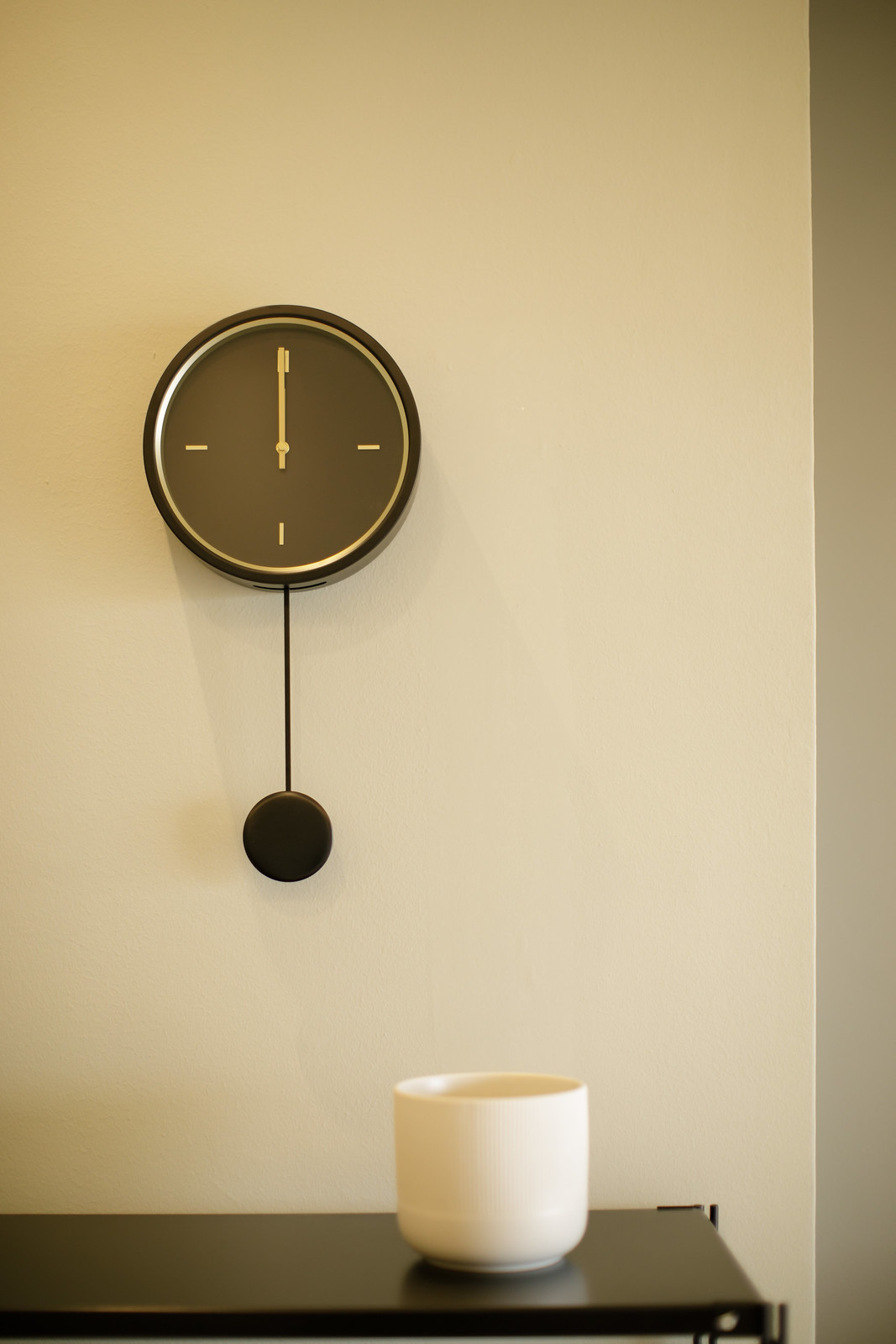In this image, we see a beautifully arranged scene featuring a clock and a tabletop. The focal point is a circular wall clock suspended above the tabletop on a light beige-gray wall. The clock stands out with its stylish design, featuring gold hour and minute hands pointing to black Roman numerals at the 12, 3, 6, and 9 positions. The clock face is bordered by a gold inner ring and a contrasting black outer ring, adding a touch of elegance. Below the clock, a black pendulum hangs from a delicate wire, adding movement and interest to the image.

Beneath the clock, a dark brown tabletop with a sleek black outer edge catches the eye. On the right side of the tabletop, there is a wide, white vase-like object, its simplicity adding to the overall minimalist aesthetic of the scene. The composition is balanced by a vertical gray strip running along the right-hand side of the wall, drawing the viewer's attention back to the central elements. The careful arrangement of these objects creates a harmonious and visually pleasing vignette.